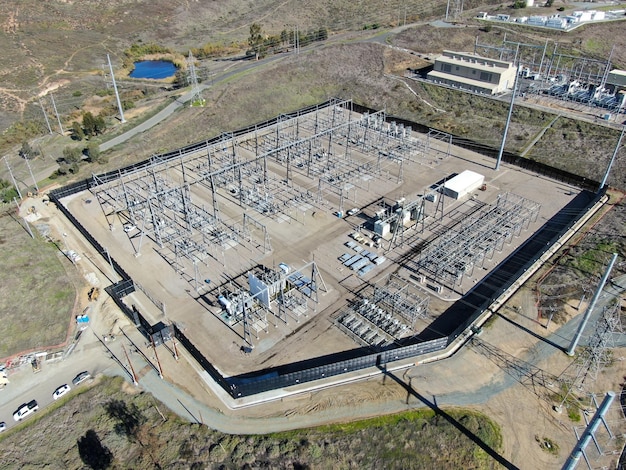This detailed aerial image, taken during the daytime in color, showcases a power station complex surrounded by vast grassland. The facility is secured by a black metal fence arranged in a mostly rectangular pattern, with a small corner cut on the lower side. Inside the fenced area are multiple generators, large metal racks, and various white buildings, including a notably large, elongated one in the far back. Several cars and trucks are parked along the entrance driveway on the left-hand side. Power lines extend from the facility up and to the right. In the top left corner of the image, outside the fenced area, there's a small pond or pool of water surrounded by foliage, emphasizing the station's remote, countryside location.